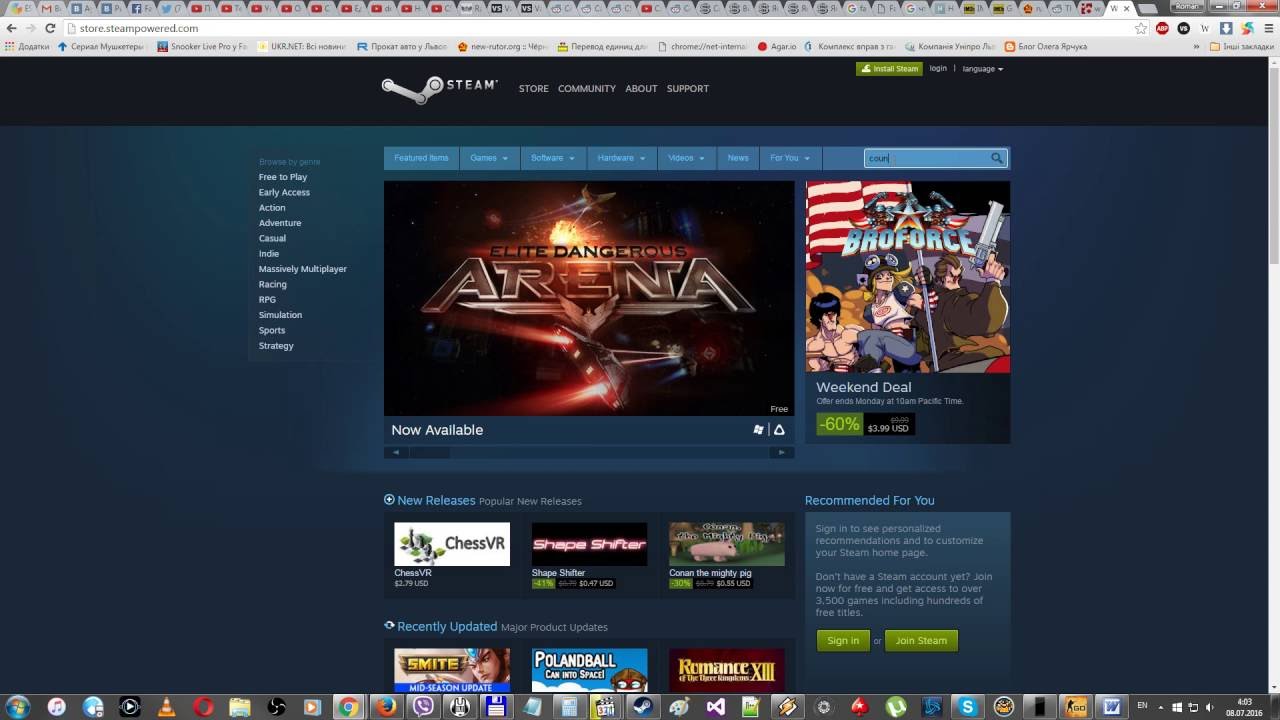The image depicts a cluttered Chrome window with approximately 30 tabs open, predominantly showing YouTube videos, alongside some Twitter and Facebook pages. The bookmarks bar is filled with numerous bookmarks, though they are too blurry to read. The active tab is on the Steam webpage, which features a black top border displaying the options: "Store," "Community," "About," and "Support." Below these, there are several indistinguishable buttons. The left sidebar lists various categories such as "Free-to-Play," "Early Access," "Action," "Adventure," "Massively Multiplayer," "Racing," "Simulation," "Sports," and "Strategy." Highlighted on the screen are elements for "Elite Dangerous Arena" and the game "Broforce."